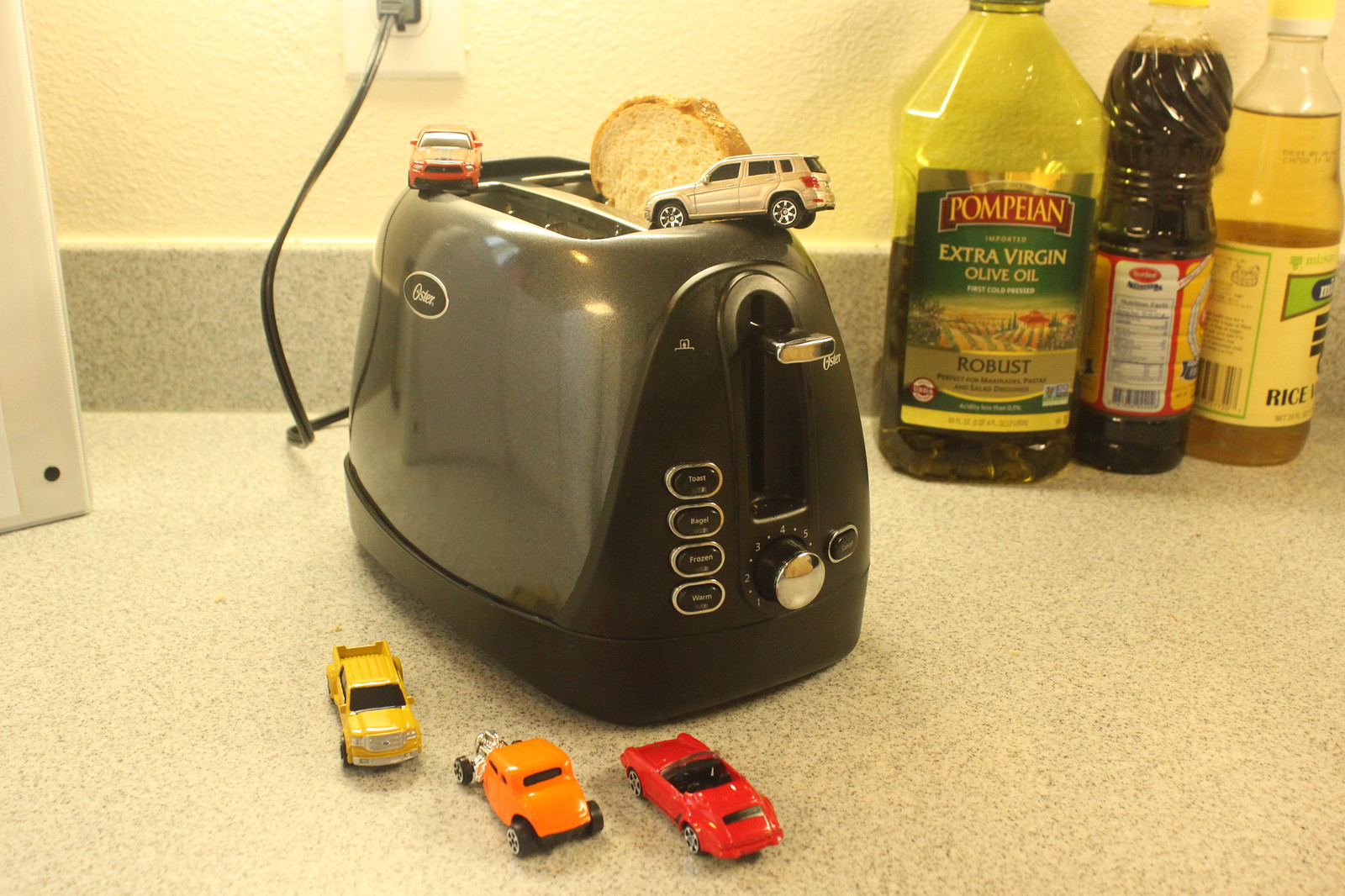The image captures a detailed scene of a black Oster toaster on a white speckled kitchen countertop against a tan off-colored wall. The toaster, which is plugged into an electrical socket, features a knob for temperature control and a lever to lower the toast. A single piece of bread is visible within the toaster slot. Perched precariously on top of the toaster are two toy cars—a tan SUV and an orange sports car. Additionally, three more toy cars—a red sports car, an orange dragster, and a yellow pickup truck—are positioned at the base of the toaster.

The background of the image includes various food items: a prominent greenish-yellowish bottle of Pompeian robust extra virgin olive oil, a container of rice vinegar, and another unidentified bottle, possibly with a brown liquid. The scene is set against a tan wall, showcasing a typical kitchen atmosphere complete with playful touches.